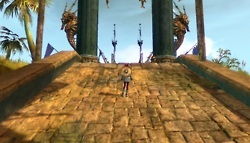In this captivating image taken from a video game, the player character stands on a weathered cobblestone ramp with their back facing the camera, sporting a large, round wooden shield securely fastened to their back. Flanking the top of the ramp are imposing green pillars, each adorned with intricate seahorse statues, lending an air of ancient majesty to the scene. The cobblestones underfoot are aged, some tinged with verdant moss, suggesting the passage of time. In the background, an expanse of clear blue sky stretches above a lush tableau of palm trees and various plants, adding a touch of tropical vibrancy to the setting. The careful attention to detail in the environment, from the texture of the stones to the natural elements, creates a serene yet adventurous atmosphere.